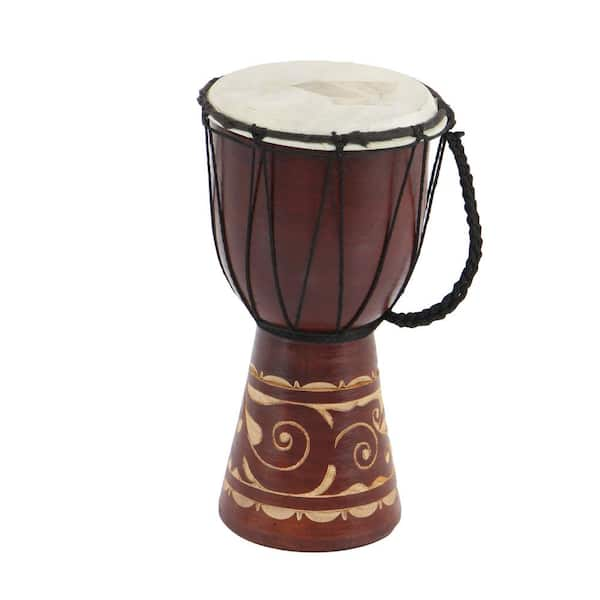The image depicts an African drum with a red-brown wooden body that narrows towards the base, creating a conical shape. The drum base features light beige painted designs that wrap around, incorporating elements like snail shapes and small flowers. The upper section of the drum is adorned with intricately tied black ropes that create decorative V-shaped patterns. Additionally, one side of the drum features a braided rope, forming a practical handle for carrying. The top of the drum is fitted with a white hide drumhead. The image is set against a clean, white background, giving it the appearance of a professional product photo with no visible shadows.